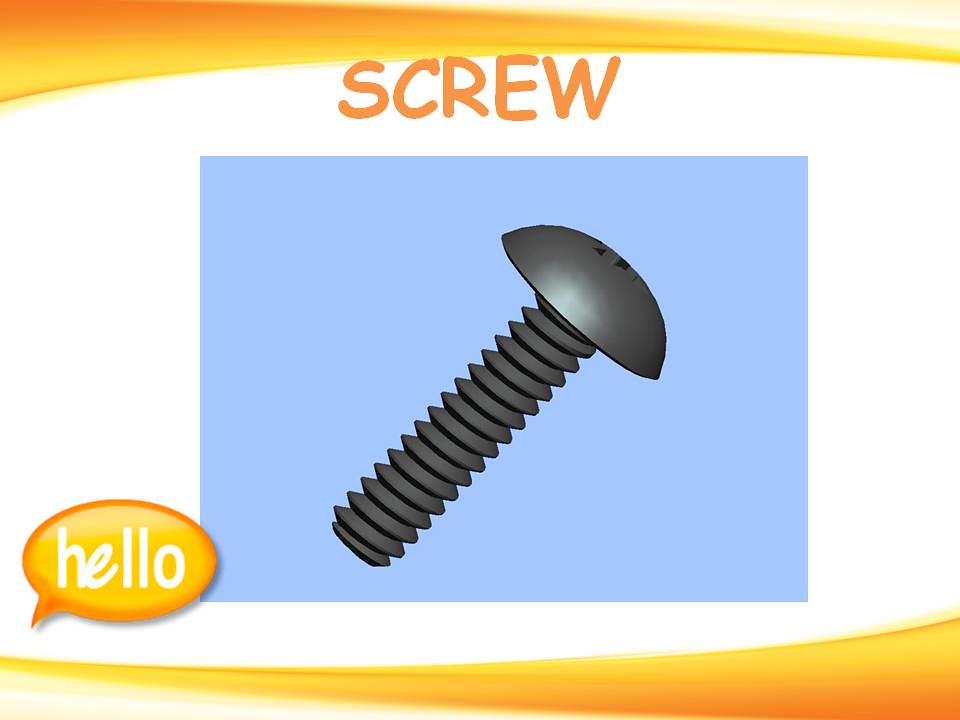The image features a detailed drawing of a dark gray screw with a rounded head and distinct threading, positioned centrally on a light blue rectangular background. The backdrop of the image is primarily white, accentuated with yellow and orange bordering lines at the top and bottom. At the top above the blue rectangle, the word "SCREW" is prominently displayed in capitalized orange letters. In the bottom left corner of the blue rectangle, there is an orange-yellow speech bubble with the word "hello" written in white lowercase letters, adding a friendly touch to the overall composition. This setup suggests that the image may be educational, potentially aimed at children to help them recognize and learn about everyday objects in an engaging manner.